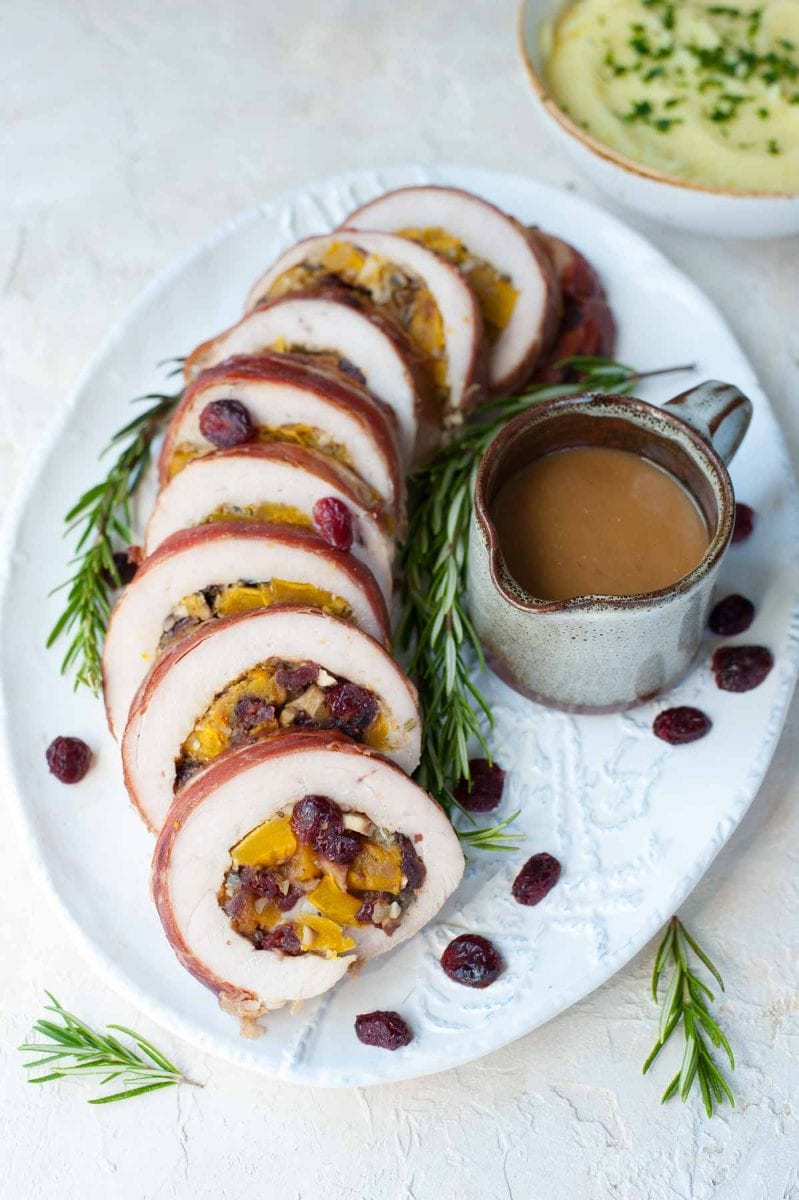This image captures an elegantly arranged plate of food in an indoor setting, likely on a white tablecloth. The focal point is a white, oval plate with embossed detailing, featuring about ten medallions of tenderloin artfully laid out in a synchronized fashion. Each medallion is layered with dried fruit, perhaps raisins or dried berries. Accompanied by the main dish is a small white pitcher containing light brown gravy. Sprigs of green herbs, possibly thyme, serve as garnish, both on the plate and the table. Behind the plate is a white bowl with a reddish rim, holding a thick yellow liquid garnished with green herbs. This well-presented dish exudes a sense of fine dining with its meticulous arrangement and complimentary garnishments.